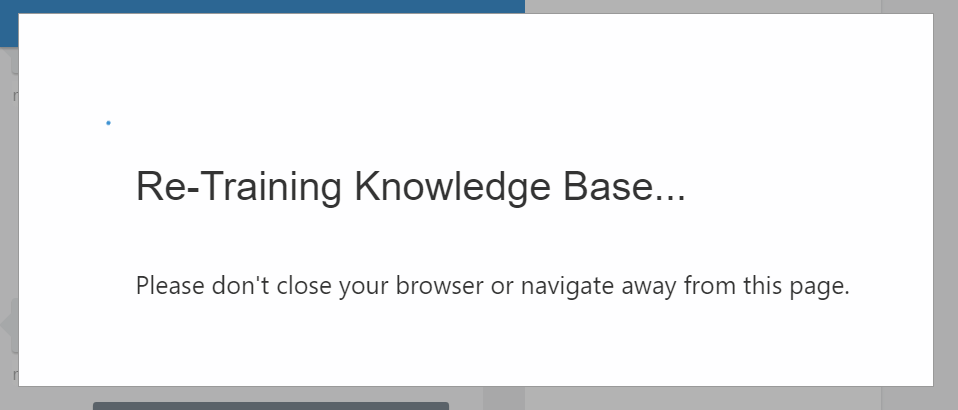This horizontally aligned rectangular image features a solid white background enclosed within a thick, mostly gray border. The border transitions to a blue color at the upper left-hand corner, extending to the top middle. The image contains two centrally positioned lines of text, both left-aligned. The top line, larger and in a dark blue or black font, reads "re-training knowledge base..." Below it, in smaller black text, the message "please don't close your browser or navigate away from this page" is displayed. Additionally, towards the bottom left of the image, there is a thin black line that extends about a quarter of the way across the page within the gray border.